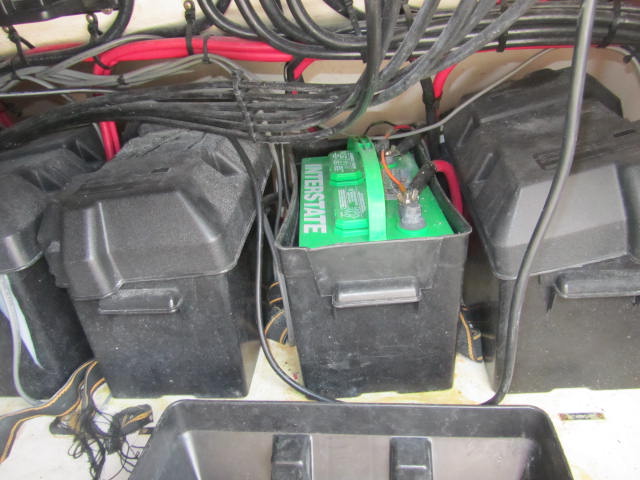The image depicts an array of interconnected black containers surrounded by a web of black, red, and gray cables. Centrally, one of the containers is open to reveal a green Interstate car battery featuring a green handle and vertical white text. The battery is ensconced in a dark gray to black plastic holder with visible cable connections on the right and additional orange wiring intermixed. To the left and right of this exposed battery, several other lidded black containers are neatly positioned, possibly indicating a series of batteries working in unison. Below the setup is a light-colored surface, further adorned with black and yellow wires and various strapping interspersed between the containers. The interconnected cables form a structured network, with some vertical, some horizontal, and others intricately bundled, contributing to a complex, organized power system.